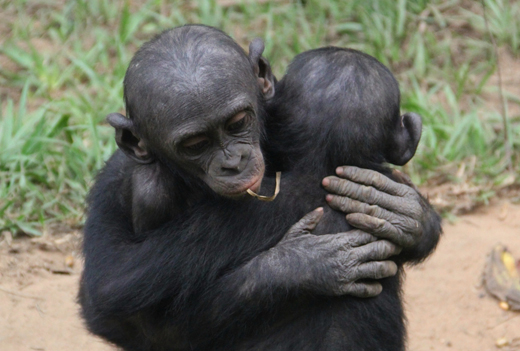The photograph captures a heartwarming scene of two young chimpanzees in a loving embrace, set in what appears to be a jungle-like enclosure. The pair, likely siblings given their similar age and size, are embraced with one looking solemnly toward the camera while the other's back of the head is visible. The chimpanzee facing the camera has a small piece of straw or grass in its mouth, adding a touch of endearing detail to the image. The chimps are covered in thin fur, particularly sparse around their heads and hands. They sit on a dirt floor with a backdrop of green, sparse grass that reveals the earthy ground beneath. The photograph, taken from a slightly downward angle, centers the chimps amidst their natural but enclosed habitat, underscoring their tender connection in this serene setting.